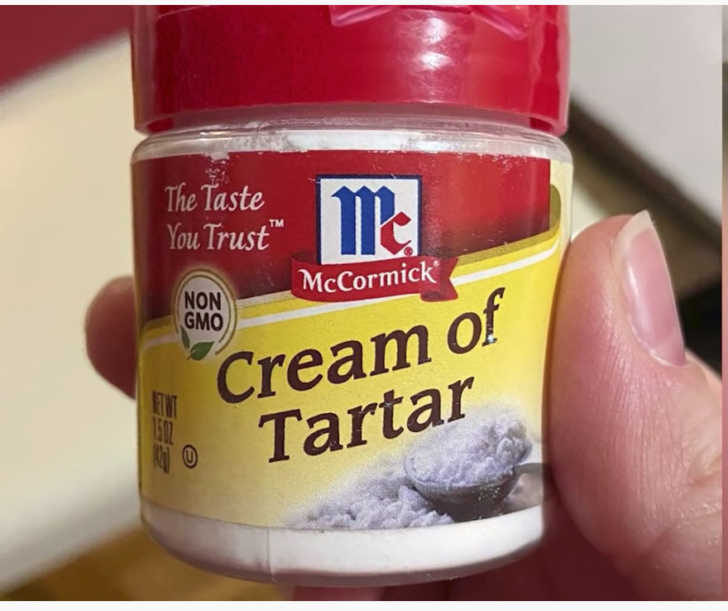In the image, a small plastic container of McCormick Cream of Tartar is held by someone's thumb and forefinger, positioned mostly centered but leaning slightly towards the top of the frame. The container dominates the image, appearing larger than life due to the close-up shot. The background is blurred, suggesting a kitchen setting, possibly near a spice cabinet.

The container features a prominent red lid, and the McCormick label is detailed with distinct design elements. The logo consists of a larger blue "M" and a smaller red "C", with a red ribbon below bearing the text "McCormick" in white. The phrase "the taste you trust" is displayed on a red background, and a non-GMO label is marked by a white circle with brown text, accompanied by two small green leaves. Further down, there are diagonal white lines on a yellow background, where "Cream of Tartar" is written in brown font. The net weight is indicated as 1.5 ounces. The container appears to show a white powder inside, typical of cream of tartar.